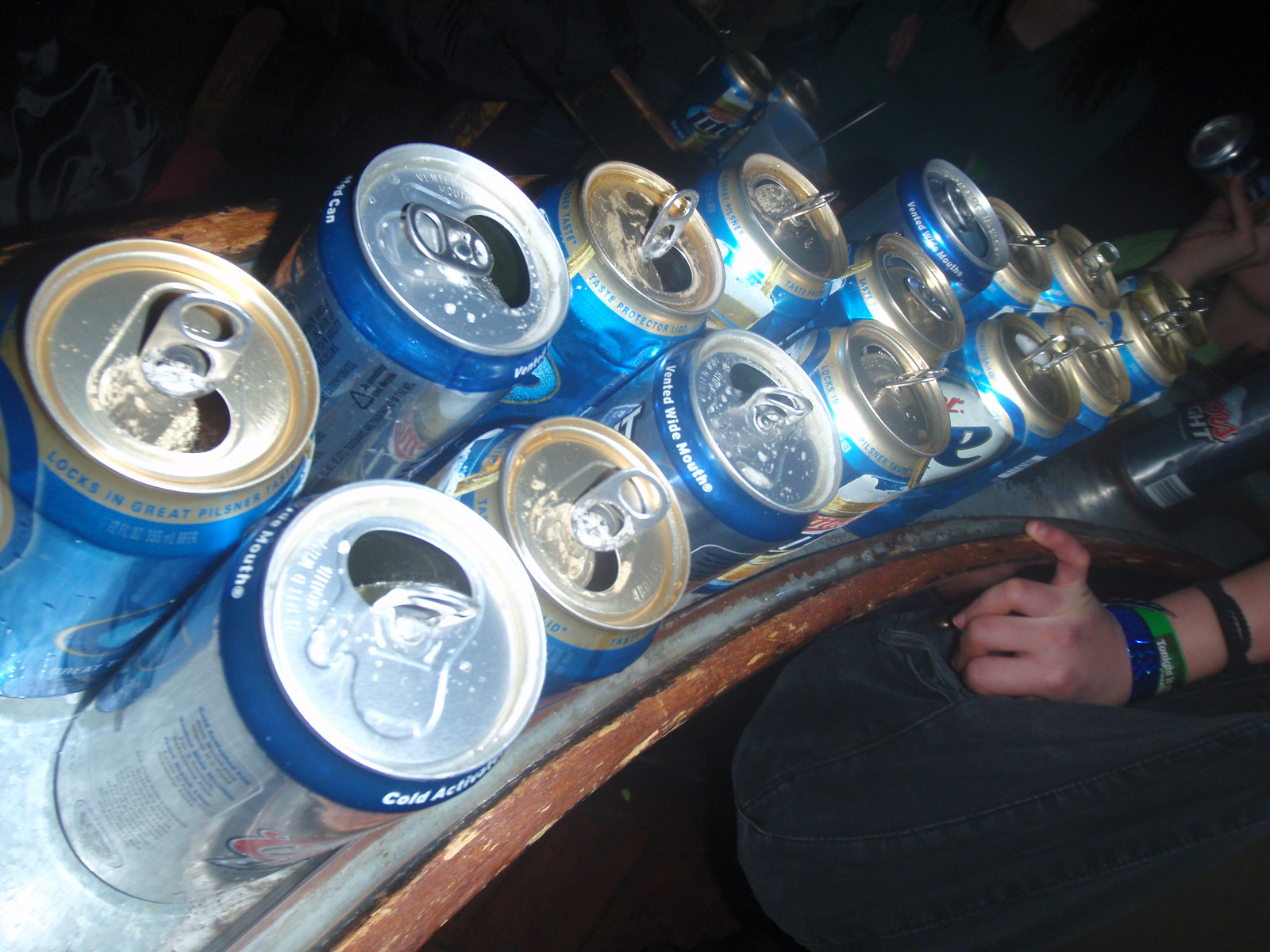In the dimly lit bar, beer cans of various brands including Coors Light, Miller Lite, Busch Lite, and Natty Lite are neatly lined up along a curved countertop. Each standard 12-ounce can is open, revealing a mix of silver and gold pull tabs, some of which are pressed back down while others stand upright. The bar's surface has a distinctive design with a white center and brown wooden edges, and it stretches from the bottom left to the right middle of the image, fully occupied by these beer cans.

In the bottom right corner, a person is partially visible with their leg and a hand resting on the counter; the hand adorned with several bracelets, including a blue one. Another individual is seen from the chin to the arm, sipping from a beer can. Further behind the bar, there is a table with two additional beer cans, one of which has the word "light" visible on it, alongside a cup with a straw. The scene hints at a lively setting, possibly a beer pong game or a casual gathering, displayed through scattered body parts of people around the scene. The lighting glints subtly off the tops of the cans, enhancing the quintessential bar atmosphere.